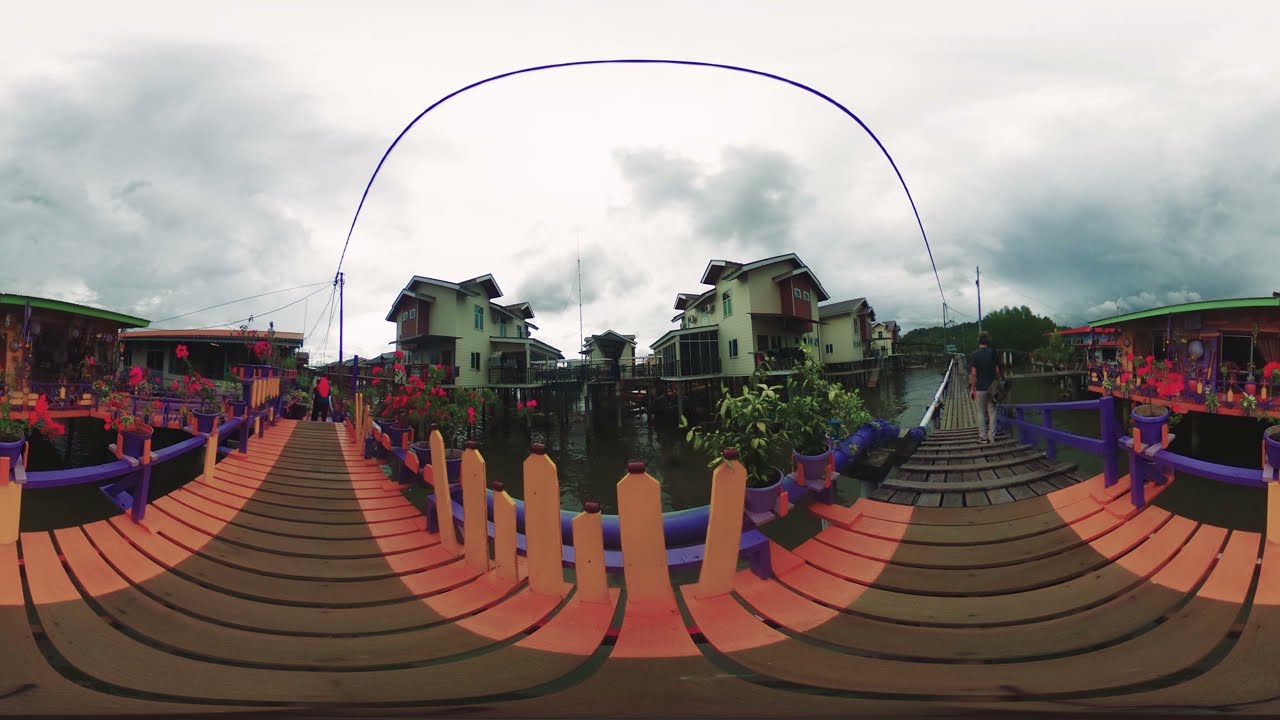The image presents an overcast, gray, cloudy sky over a picturesque seaport town, captured with a fisheye lens that creates a distorted, panoramic view. Central to the scene is a pair of interconnected boardwalks, meeting at a rounded U-shaped fence. The boardwalk itself consists of brown wood with red and orange or salmon-hued borders. Flanking the boardwalk are purple wooden railings and a series of blue and black pots containing blooming roses. To the side, one notices a striking blue thin wire extending across the scene. The town features multiple yellow-sided, stilt-supported buildings beside the dark gray water. In the distance, lush green trees are visible. Painted brown with peach accents, the bridge along the boardwalk offers a path for individuals to traverse, contributing to the tranquil yet bustling atmosphere of the seaport. In the background, residential buildings rise, accompanied by small shacks and a person walking along the bridge, adding a sense of scale and life to this detailed coastal snapshot.